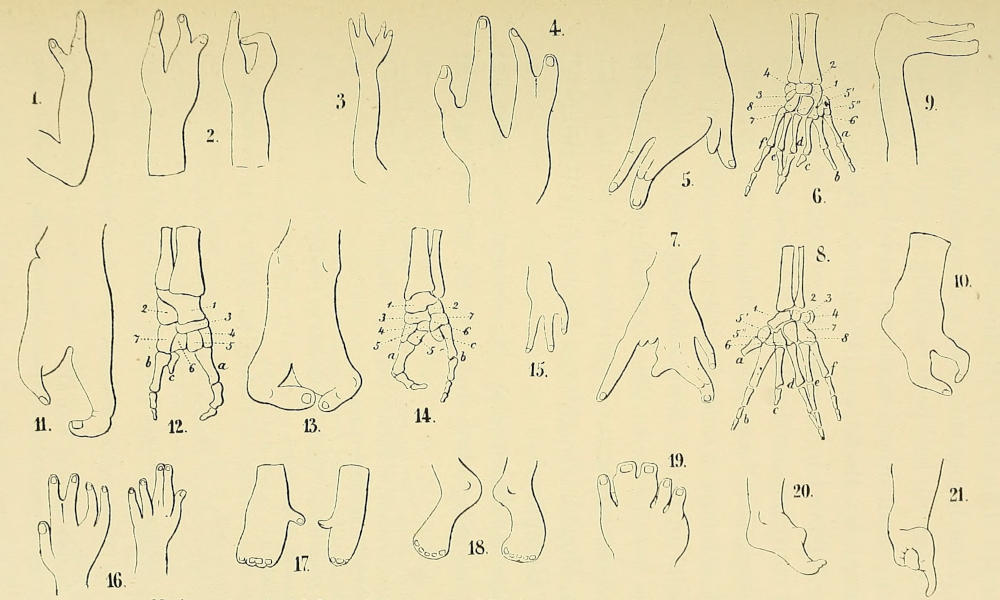The image displays 21 detailed line drawings against a yellow background, showcasing various appendages, including arms, hands, and feet, illustrated in a blue or black ink. Each illustration appears to depict different forms of deformities or anomalies. The series starts with an arm bent at the elbow with its forefinger and thumb pointing upwards and continues through to the 21st drawing. Many of the hands are drawn with fingers bent in unnatural ways or with an unusual number of fingers, ranging from two to four or fused together. Some drawings represent skeletal structures of hands, highlighting bones and joints. One image, in particular, appears to depict a hand resembling a duck. The feet are also shown with fingers fused together. Overall, these illustrations seem to be studies or concept sketches, possibly from a medical journal, illustrating various abnormalities of human extremities.